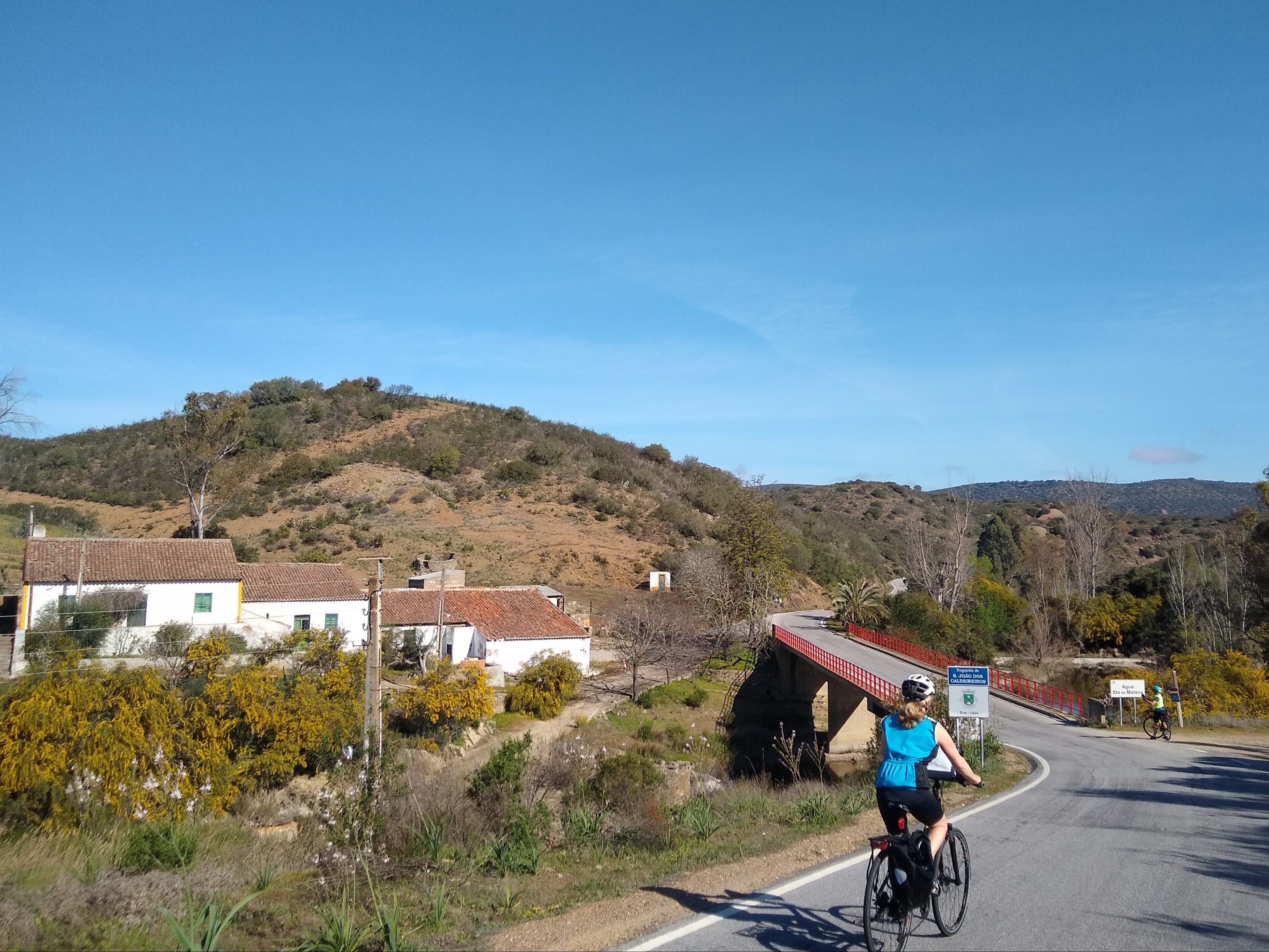The photograph captures a serene wilderness scene featuring a picturesque small town. In the foreground, a woman with blonde hair tied in a ponytail is cycling on a black bike. She is dressed in black pants, a blue vest or tank top, and a white helmet. She approaches a left turn onto a bridge with red railings. Ahead of her, another cyclist in a yellowish shirt is visible but at a considerable distance. To the left of the roadway, several white buildings with Spanish-style red ceramic roofs can be seen, possibly houses or repurposed structures. The road runs parallel to what appears to be a river, which is partially visible beneath the bridge. The landscape in the background is characterized by brown, rolling hills dotted with low bushes and brush, contributing to a dry, almost desert-like atmosphere. Scattered near the river, a few trees break the otherwise open and vast environment. The scene is bathed in natural light under a clear, expansive blue sky.